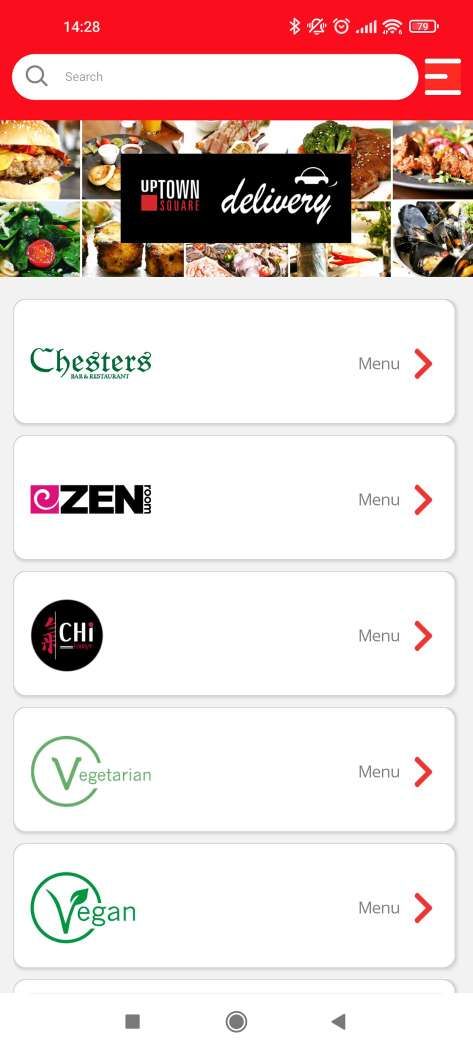This is a detailed screenshot of a mobile application interface. The app features a vibrant red header at the top. In the upper left corner, the time is displayed in white as "14:28," while the upper right corner houses several icons. Directly below the header is a sleek white search bar, designed as an elongated pill shape. On the left end of this search bar, there is a medium gray magnifying glass icon, indicating the search function. Beside it, in small light gray text, the word "Search" is displayed. Adjacent to the search bar on the right side, there is a white hamburger menu icon, with the center white line shorter than the top and bottom lines.

Beneath these elements, there is a header image that consists of a collage of various food photographs. The collage is neatly segmented into five images per row, arranged in two rows, each image separated by thin white lines. At the center of this collage, there is a prominent black rectangle. Within this rectangle, positioned in the top left corner, the word "uptown" is written in white, with "town" appearing taller but with the top of the text aligned. Below this, the word "square" is displayed in red text right under "town." To the left of this text, a red square visually fills the remaining space. On the right side of the rectangle, in elegant white cursive text, the word "delivery" is written, and slightly upwards and to the right of it, there is a cartoon-style white car icon.

Underneath the collage, the background transitions to a light gray shade. This section contains various interface elements, represented as white rectangles with rounded corners. These panes are separated by a small amount of negative space and cast subtle medium gray shadows on the background. Each pane has a title on the left side, with the word "Menu" in light gray text to its right. To the far right of each pane, there is a bright red arrow, indicating a clickable or navigable element.